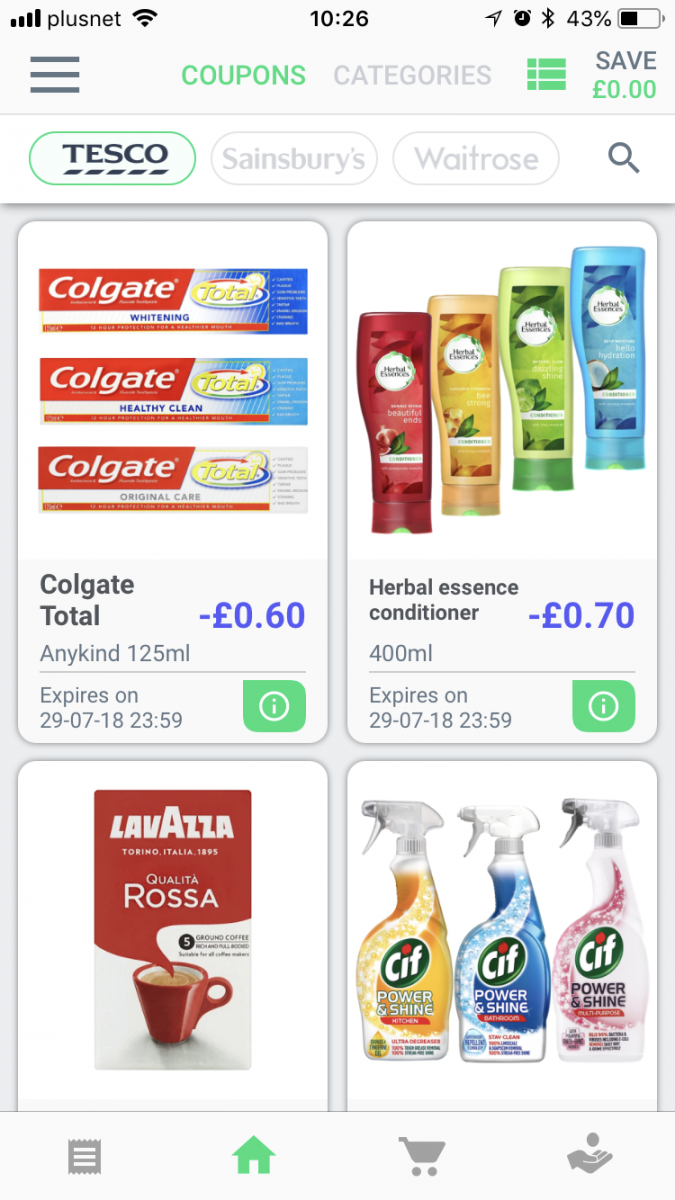The page showcases various special offers from Tesco, highlighting savings that can be achieved using coupons. 

- **Colgate Total Toothpaste (125ml, any kind)**: Save 60p. Offer expires on July 29th.
- **Herbal Essences Conditioner (400ml)**: Save 70p. Offer expires on July 29th. 

Additionally, there are offers on Lavazza Qualità Rossa Coffee and three varieties of Sif cleaning products. Unfortunately, the bottom of the page is not fully visible, so the savings details for Lavazza and Sif are not shown.